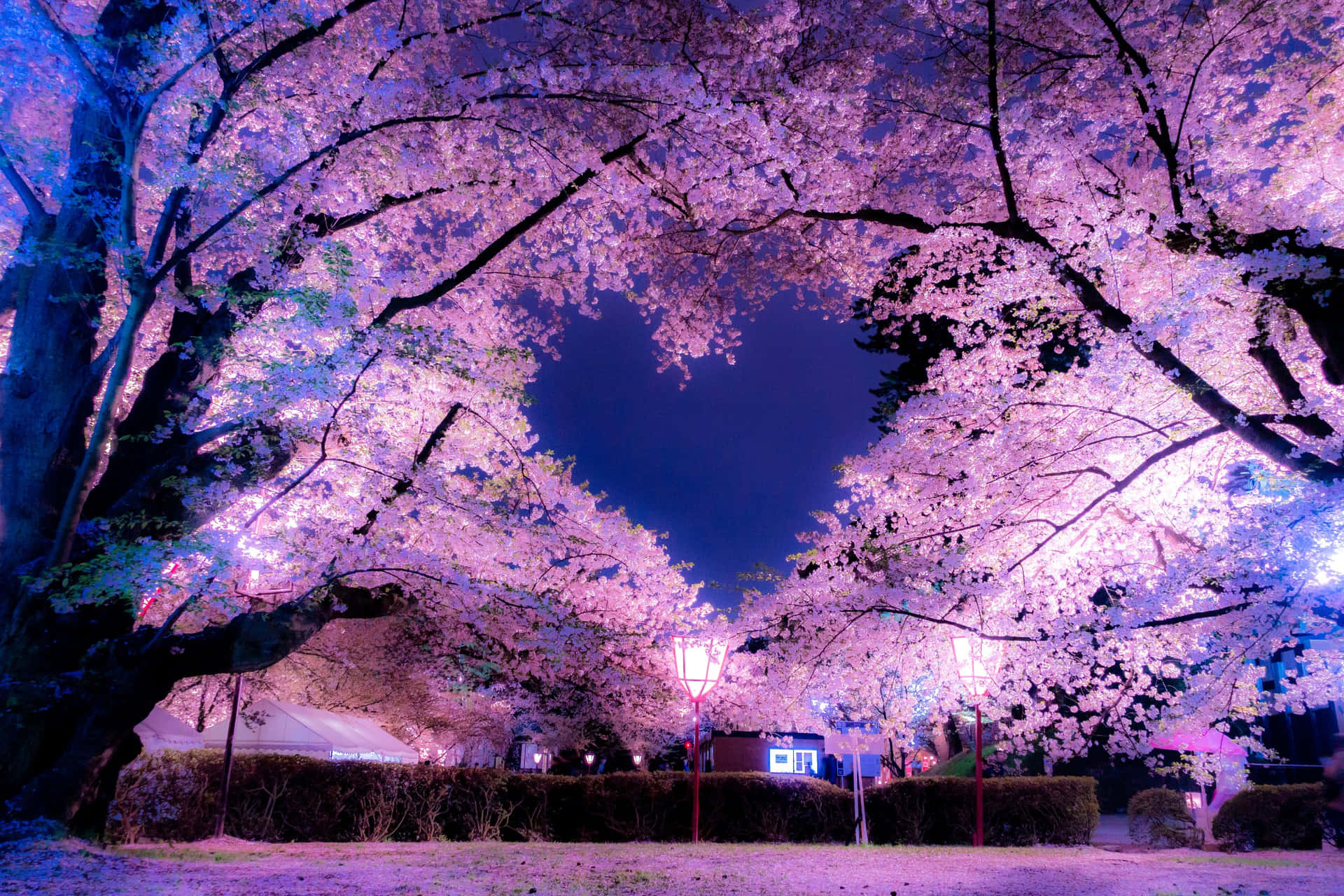The image captures a serene early evening or nighttime scene in an open courtyard. The sky overhead is a deep midnight blue, still showing traces of twilight with a touch of blue. Set against this backdrop are blooming cherry blossom trees with large, arching branches covered in light lavender and pink flowers. These branches interlace above, forming an enchanting heart-shaped opening to the sky. Below, the ground is carpeted with fallen petals, creating a soft, pastel blanket in hues of white, lavender, and pink. Flanking the courtyard are two tall lampposts, possibly red or pink, casting gentle light that enhances the romantic ambiance. Among the highlights, two or three buildings are visible in the background, and there might be a garden umbrella in pink or purple. The scene is further bordered by a line of bushes and hedges, adding a tinge of green to the picturesque setting.